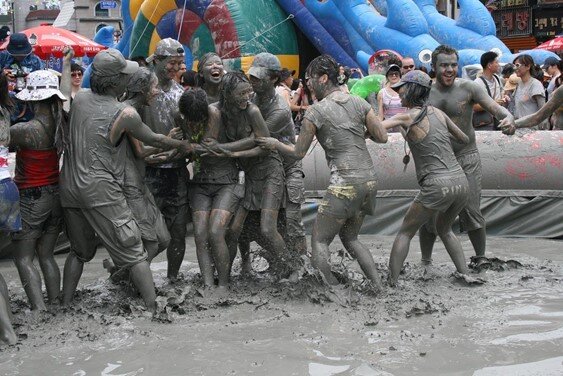This photo captures a lively scene at an outdoor festival, likely in South Korea, where a group of around ten college-age participants, both men and women, are enthusiastically engaged in a mud fight within a large inflatable pool filled with dark grey mud. The participants, dressed in casual athletic wear, including shorts and t-shirts, are completely covered in mud as they splash and throw it at each other, clearly reveling in the messy fun. Behind the mud-soaked festivities, a crowd of onlookers, who are noticeably cleaner, watches the spectacle with amusement. The background features a vibrant mix of inflatable structures in various colors, a red-canopied carousel or tent, an inflatable water slide, and umbrellas branded with a soda company’s logo. Adding to the festival atmosphere, signs in Korean, including one for "Noraebang" (karaoke), provide a cultural touch, while the city’s buildings rise in the distance, framing this exuberant urban celebration.